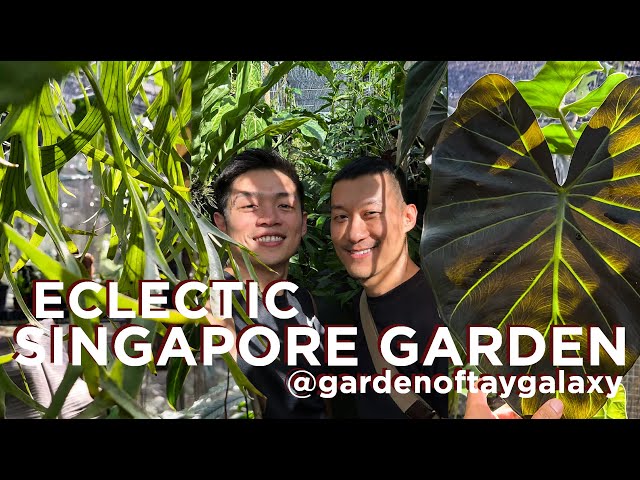The image is an advertisement poster featuring "Eclectic Singapore Garden at Garden of Tay Galaxy." The backdrop consists of black bars at the top and bottom, framing a lush, tropical setting filled with a variety of plants, including tall grasses, trees, and a massive green elephant ear leaf on the right. In the center of the poster, two Asian men are smiling directly at the camera. The man on the left is dressed in a black T-shirt with a strap across his chest, likely holding a bag, while the man on the right wears a suit coat, white shirt, and tie. Both have short, dark hair and are partially obscured by the dense foliage surrounding them. The text "Eclectic Singapore Garden at Garden of Tay Galaxy" is written in white, positioned prominently at the center of the image.